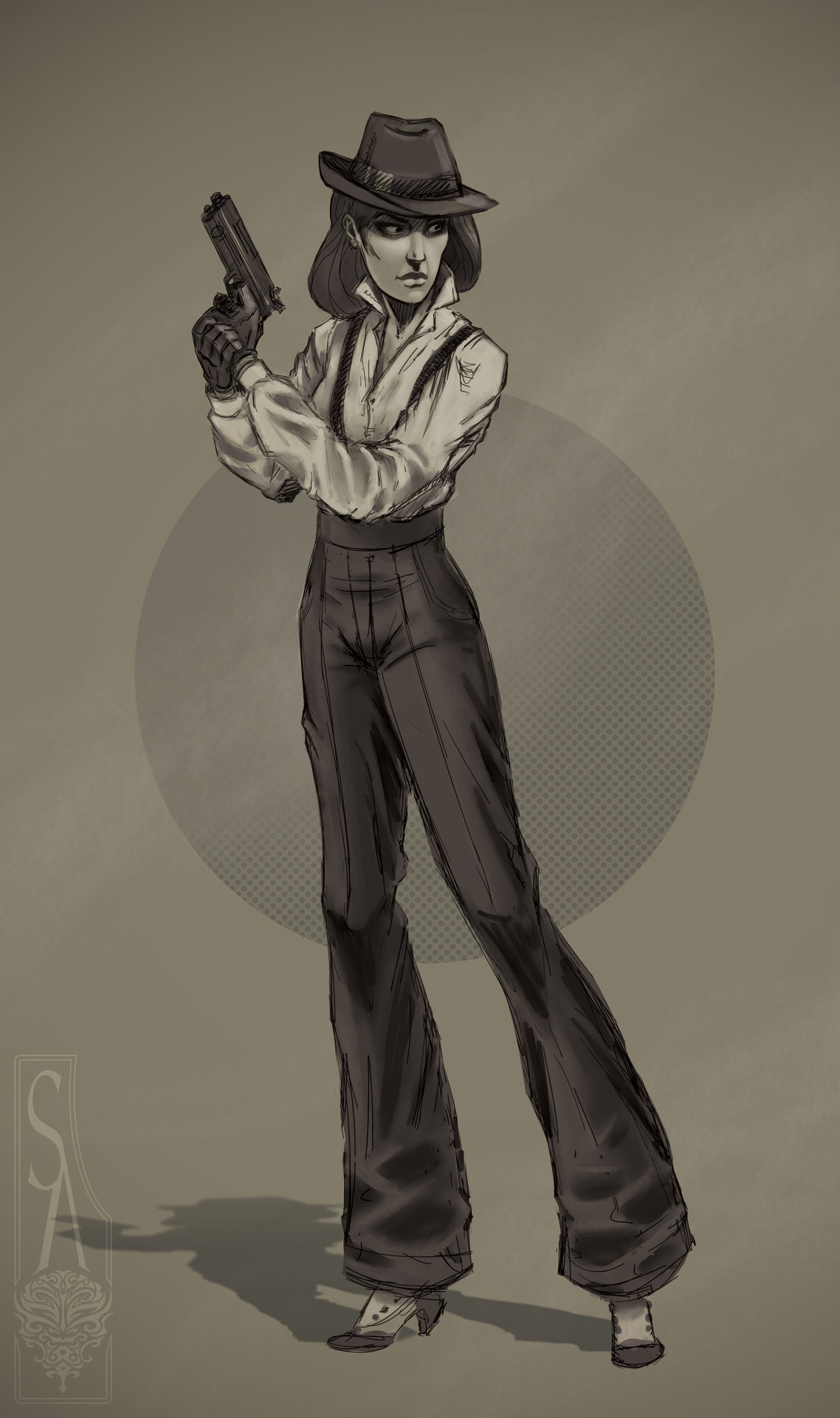This image is a detailed, digitally-drawn illustration of a tall woman in a black-and-white, noir-style setting. The character, portrayed in a cartoon style with pencil lines, is reminiscent of a detective. She wears a fedora hat over short hair, black gloves, and a white collared button-down shirt with suspenders. She holds a black pistol in both hands and is dressed in long black pants paired with high heels. The background is a gradient of gray tones, featuring a darker gray circle in the middle. In the bottom left corner, the lettering "SA" appears alongside a small graphic logo.